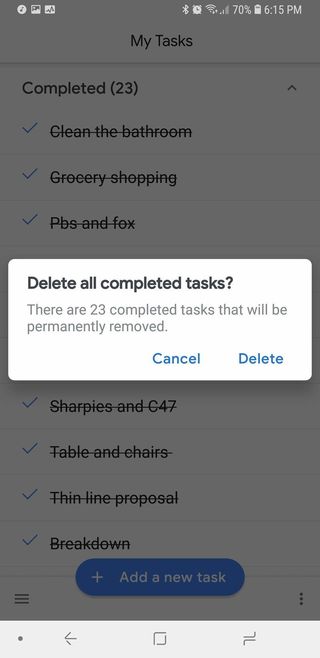The image displays a smartphone screen, specifically an Android device, showcasing a task management application called "MyTasks." The primary screen reveals a background filled with a list of various tasks that have already been completed, each item marked with a checkmark and a strikethrough line. The tasks visible in the background include "Clean the bathroom," "Grocery shopping," "PBS and Fox," "Sharpies and C-47," "Tables and chairs," "Thin line proposal," and "Breakdown," among others.

A dialog box is prominently displayed at the center of the screen, partially obscuring the task list. The dialog prompts the user with the message: "Delete all completed tasks. There are 23 completed tasks that will be permanently removed." The user is given two options: "Delete" or "Cancel." Below the dialog, a blue button labeled "Add a new task" is situated at the bottom, inviting the user to add more tasks if needed.

The user interface design is clean, with a predominantly white background providing a clear contrast to the text and interactive elements. The top notification bar indicates the current time, 6:15 PM, with the battery level at 70%. The bar also shows an alarm icon, Bluetooth connection status, and several other app notifications, including one that seems to be related to music and another that resembles a stock market graph.

Overall, the image effectively captures the state of a completed task list within the MyTasks app, accompanied by the option to delete all finished tasks for a clean slate.